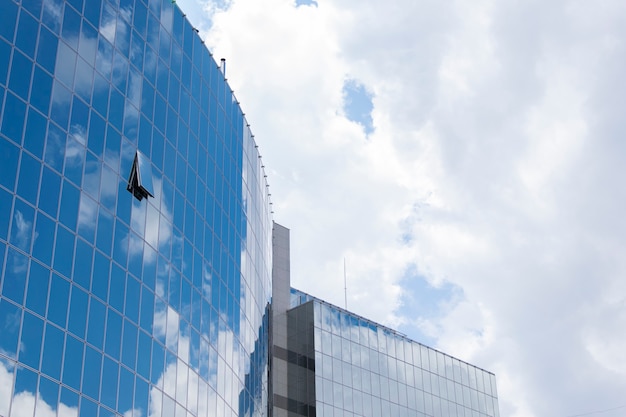The image captures an upward view of a complex architectural scene dominated by two skyscrapers. Both buildings are entirely clad in mirrored glass windows that vividly reflect the blue, cloud-filled sky. One building, positioned on the left side of the frame, features a distinctive curved design, transitioning smoothly into the adjacent, more rectangular structure. The latter building occupies the right middle section of the photo. A single window in the curved building is propped open from the bottom, hinged at the top, and is located in the middle of the building on the left side. The scene includes a hint of a concrete structure between the two buildings, adding an additional layer of depth. The sky above is extensively occupied by two enormous clouds, creating a dynamic backdrop that is beautifully mirrored on the building's glass surface.